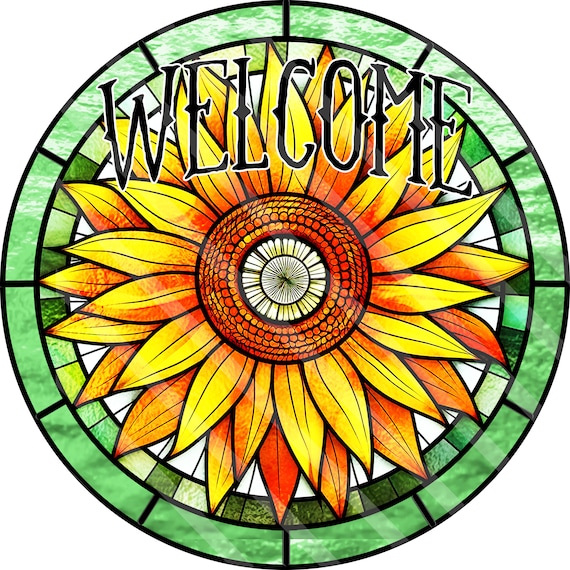The image is an illustration designed to mimic a stained glass window that features a welcoming motif. At the top of the image, "WELCOME" is boldly written in black text. This circular stained glass pattern is framed with a border resembling green stained glass, varying in shades from dark to light and marbled. Central to the image is a large, vibrant sunflower with layers of pointed yellow and orange petals radiating outward. The core of the sunflower is densely packed with tiny white petals interspersed with an orange scaly texture. The background behind the sunflower consists of white and black textured glass, adding depth and contrast to the vibrant colors of the flower. This piece appears to be an artistic representation suitable for display in one's home.